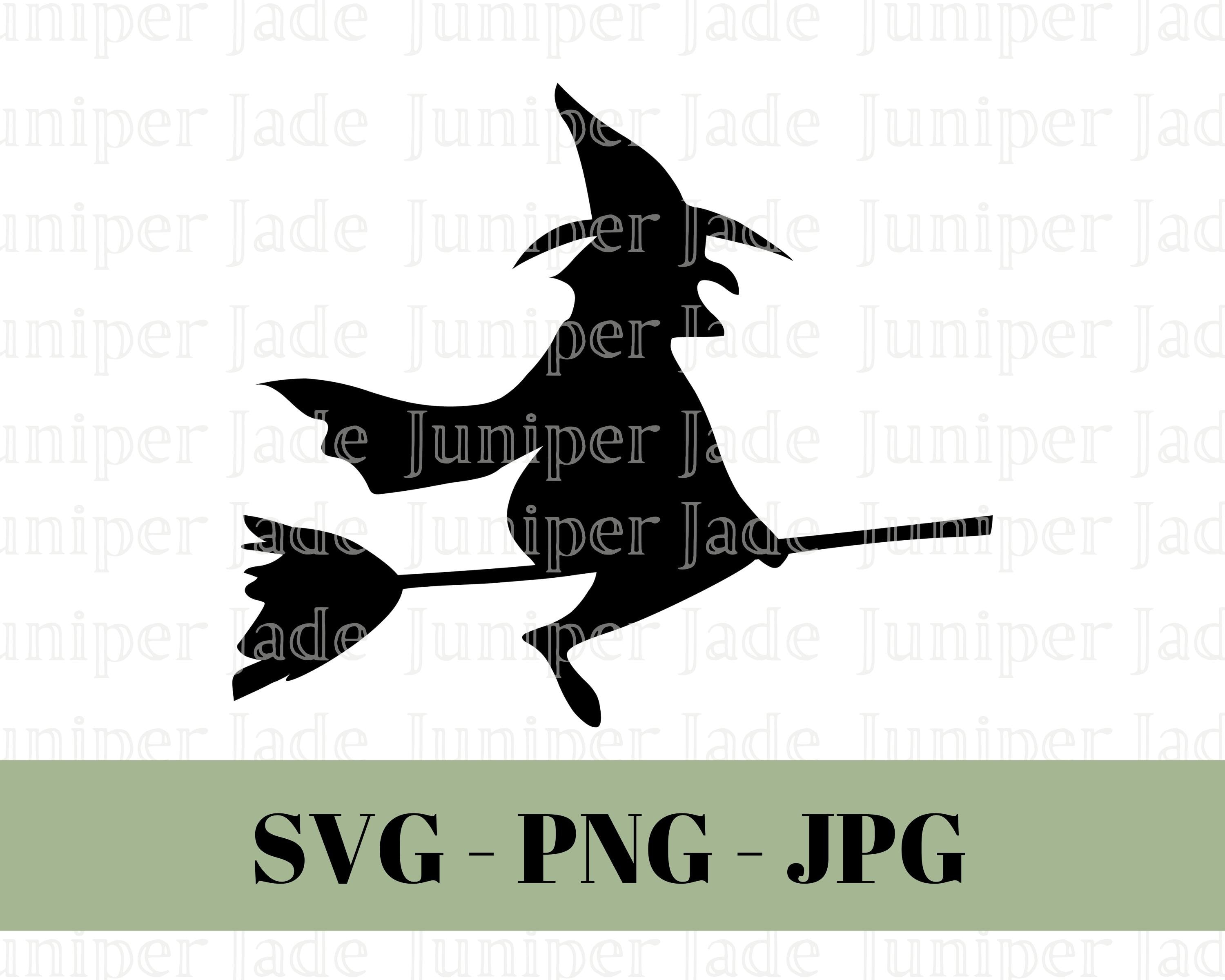This image features a silhouetted, all-black witch with a pointed hat, a long pointy nose, and a pointed chin, riding a broomstick and flying to the right. The witch is adorned with a flowing cape. Overlaid across the entire silhouette in repeating horizontal lines is a watermark that reads "Juniper Jade" in lighter text. Below the witch, there is a light green banner displaying the text "SVG-PNG-JPG" in dark, bold, all-capital letters. The background of the image is predominantly white, emphasizing the contrast of the silhouette and the overlaying details.